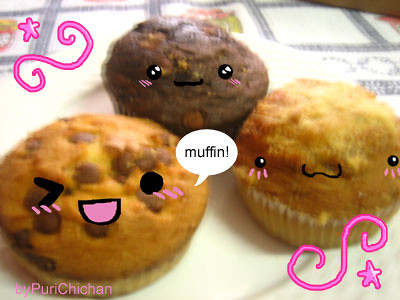This image depicts an edited photograph of three muffins on a white ceramic plate set atop a table with a quilted, square-patterned tablecloth, suggesting a cozy home setting. The muffins are designed with cartoonish, anime-like faces, including blush on their cheeks and varying expressions. The muffin on the bottom left is a vanilla muffin with chocolate chips and has a winking eye and an open mouth. The chocolate muffin in the back displays two open eyes and a small smile. The muffin on the bottom right, possibly a vanilla or streusel muffin, has wide eyes and a cheerful grin. Surrounding the image are decorative elements like pink squiggly lines, stars, and a dialogue bubble with the word "Muffin!" in it. The artist's watermark, "by Puri Chichun," is also present.